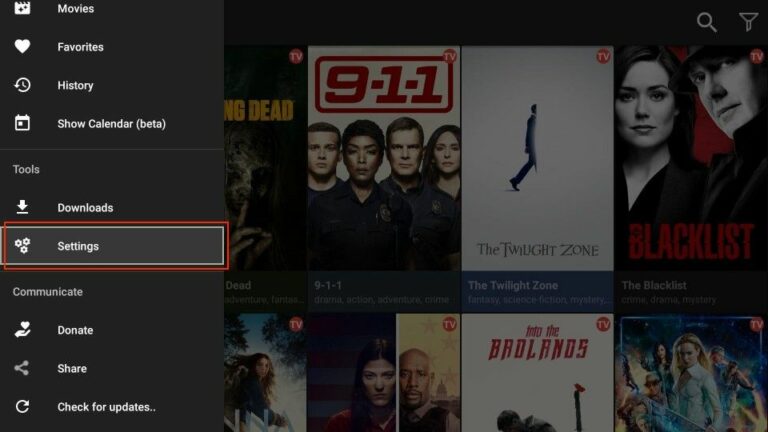This screenshot captures a multimedia interface detailing various sections and icons dedicated to media management and content access. On the left-hand side, there is a vertical menu featuring a series of black boxes labeled with white text. At the top of this menu, the section titled "Movies" includes its corresponding icon. Below, there are icons and labels for "Favorites" (indicated by a heart icon), "History," "Show Calendar," and a "Beta" tag. Further down, the "Tools" section comprises options like "Downloads" and "Settings," the latter of which is prominently outlined in red.

Additionally, the "Settings" box contains sub-options such as "Communicate," "Donate," "Share," and "Check for Updates." Spanning the main content area are images of various TV series and films available on CDs. Notable titles include "9-1-1," "The Twilight Zone," "Badlands," "Blacklist," and "The Walking Dead." Each CD cover is accompanied by a small TV icon in the upper right corner signifying content that has aired on television. While several titles are partially obscured, these are the identifiable ones. The interface appears to be a comprehensive tool for managing and accessing a curated collection of video content.